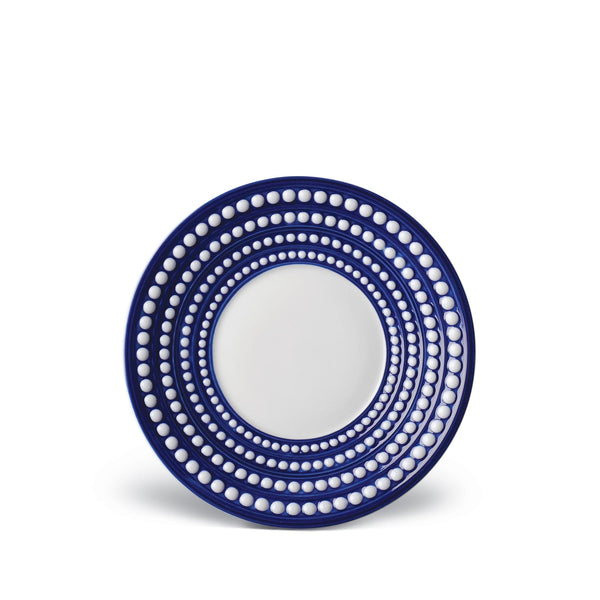The image showcases a round, dark blue dinner plate standing upright against a white background. The plate features a large, white circular center. Surrounding this center are four concentric rings of white dots that increase in size as they approach the outer rim. The plate appears to be textured, with the white dots potentially raised above the surface. A shadow beneath the plate adds depth to the otherwise minimalistic composition.